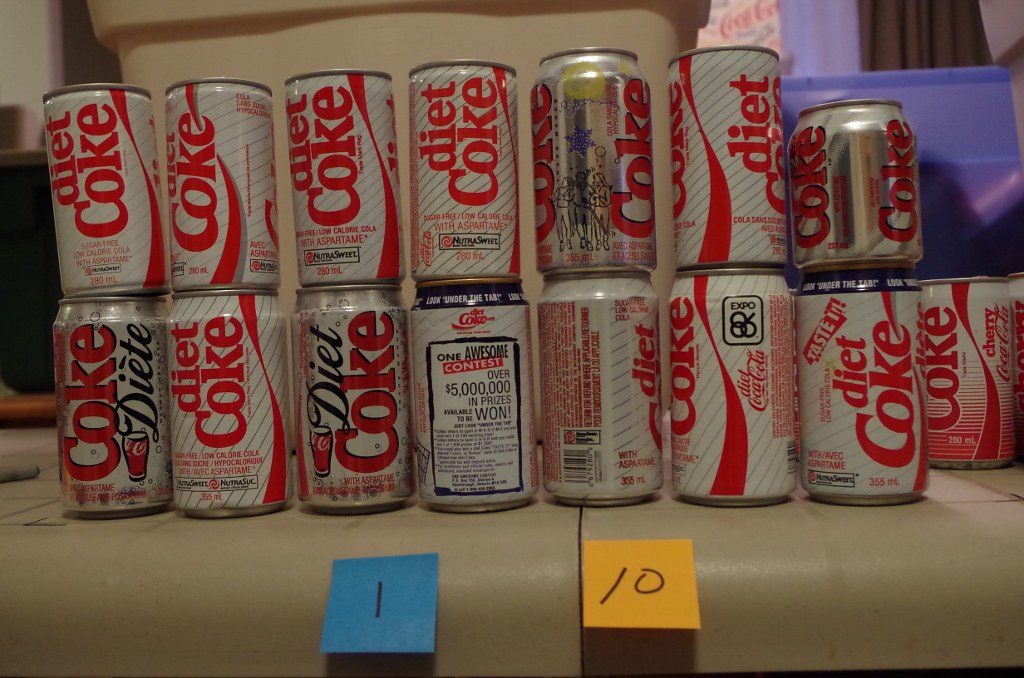The image showcases a meticulously arranged display of soda cans on a slightly glossy, tan-colored stage that is elevated from the rest of the scene. Behind this platform, there is a background consisting of tan and purple plastic components, possibly tote bins or panels. 

On the tan floor in the foreground, a blue post-it note marked with the number "1" and an orange post-it note marked with the number "10" are prominently placed. Dominating the display are various Diet Coke cans. The top four or five cans share the same design, featuring a white background with red "Diet Coke" branding and a distinctive swirled stripe pattern. Below them, two cans stand out with their shiny aluminum surfaces, reflecting light more prominently. These cans feature the word "Diet" in black and "Coke" in red.

To the right of this main arrangement, there are two or three additional varieties of cans. A couple of these replicate the design of the initial white and red cans, while the remaining ones include a shorter silver can and another bright silver can, differing from the white and red theme. The entire setup appears well-organized and curated, highlighting the different packaging designs of Diet Coke.